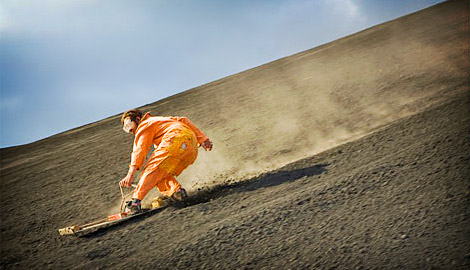This image captures a man dirtboarding down a steep, dark brown, sandy embankment, surrounded by a dusty plume trailing behind him. He’s dressed in an orange jumpsuit and clear goggles with a white strap, shielding his brown hair and focused gaze. His makeshift wooden board, equipped with a handle, allows him to maneuver as he crouches with one knee bent, feet securely strapped in. The light of day casts a long shadow, indicating late afternoon under a blue sky dotted with a few clouds. He moves swiftly down the slope from the top right toward the bottom left of the frame, exuding a dynamic sense of action and adventure.